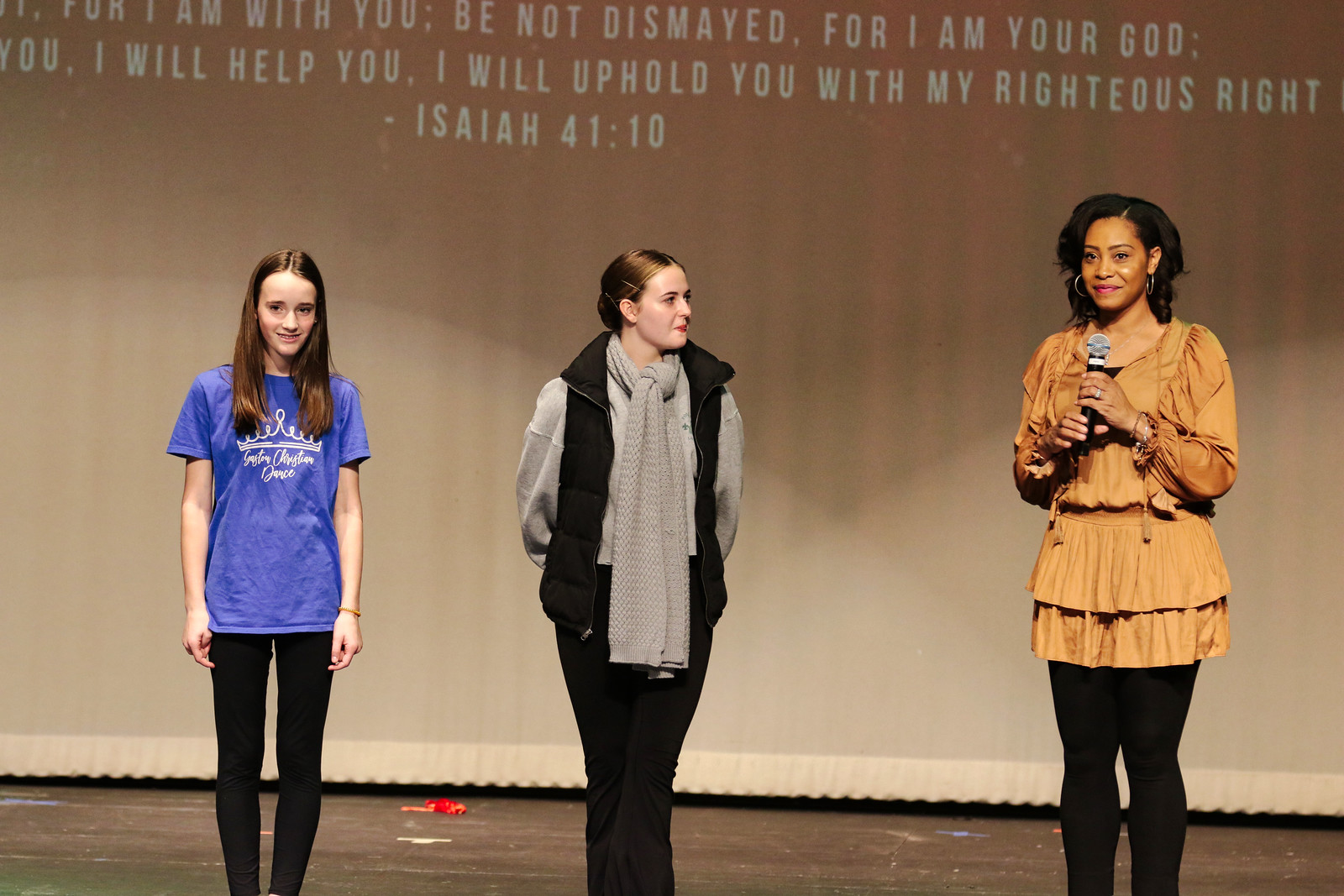In the image, three individuals stand on a stage, aligned from left to right, against a backdrop featuring the Bible verse Isaiah 41:10, which reads, "For I am with you, be not dismayed, for I am your God. I will help you, I will uphold you with my righteous right hand."

On the left is a young girl, possibly a preteen or teen, with long brown hair cascading over her shoulders. She is dressed in a blue t-shirt with white writing and black leggings. She looks straight ahead and smiles faintly.

In the center stands a woman with short brown hair styled in an updo. Clad in a gray shirt encircled by a long bow from her neck to below her waist, a black vest, and black pants, she looks towards the woman on her left.

The woman on the far right, clearly the central figure, appears to be the lead presenter. She is an African American woman, holding a microphone in both hands, dressed in a vibrant yellow top and black leggings. Her dark hair is complemented by large hoop earrings, and she wears a warm smile as she looks out towards the audience.

The stage setting and the attire suggest a formal event, possibly a church gathering or a presentation similar to a TED talk, held during the cooler seasons of fall or winter.